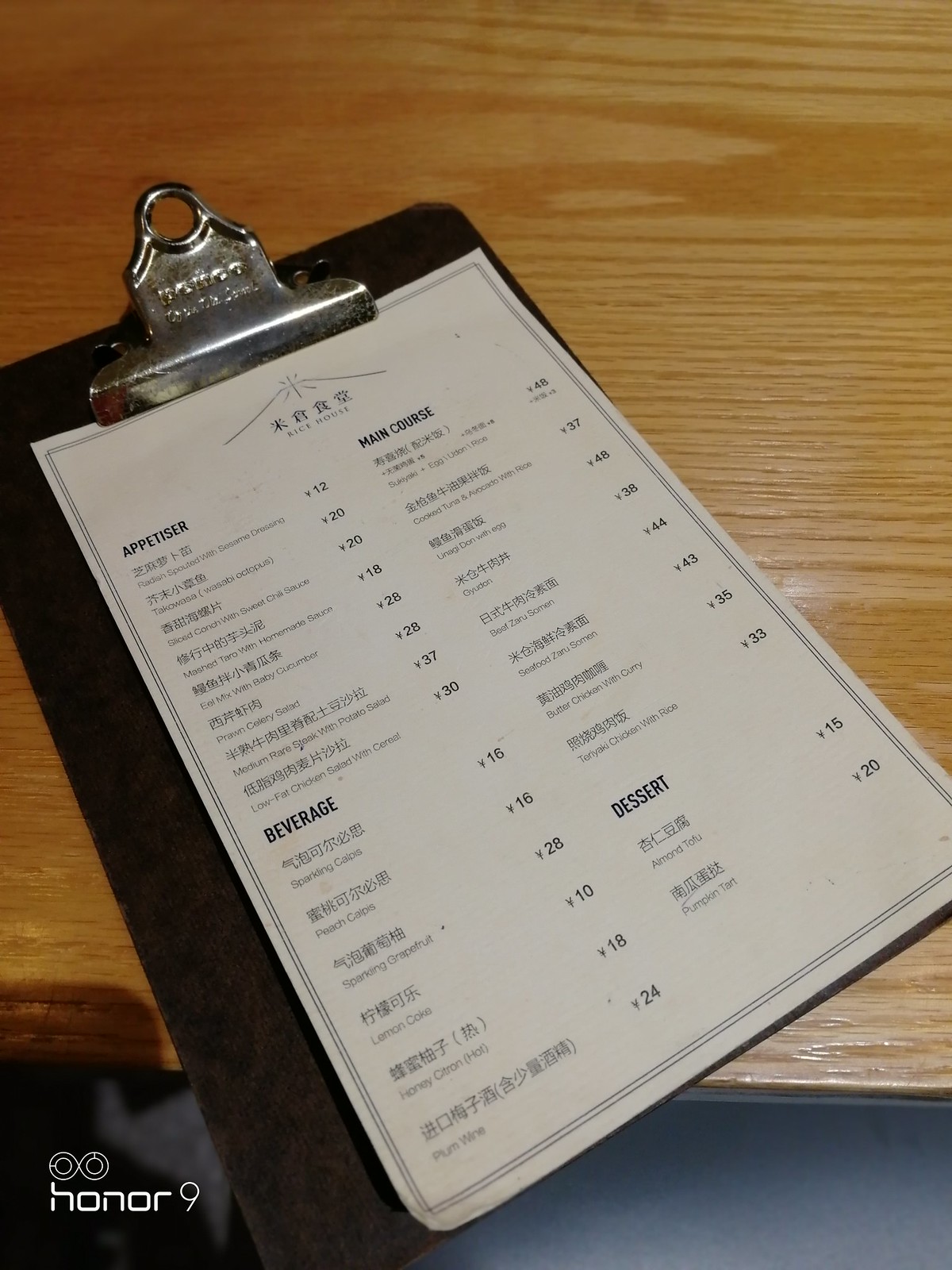In the image, a dark brown clipboard holds a restaurant menu. The menu, securely attached to the clipboard, features distinct sections for appetizers, beverages, main courses, and desserts. The clipboard itself rests on a light brown wooden table. Below the table, the background is a light grayish hue. In the lower left corner of the image, the text "Honor 9" is visible alongside a horizontally oriented figure 8. While the menu items are listed in a non-English language, some of the prices are discernible, with numbers such as 12, 20, 18, 28, and 29 clearly visible.